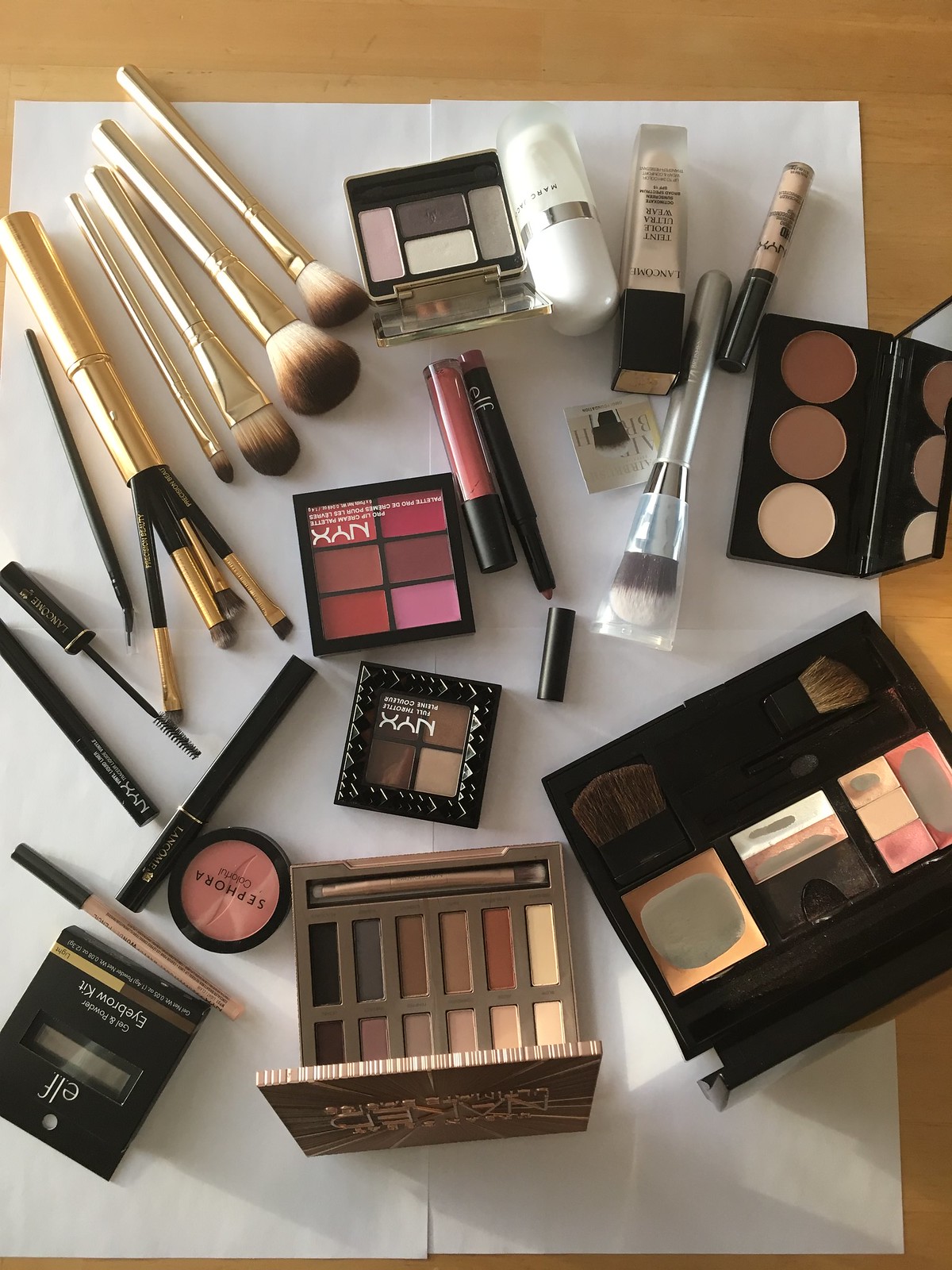The image depicts a light-toned wooden table showcasing a distinct wood grain pattern. Laid out neatly on the table are white papers arranged in a grid of four squares, serving as a backdrop for a variety of makeup products and tools. 

In the top left section, there are nine different makeup brushes, ranging from eyelid to blush and powder brushes. Each brush features gold trim with bristles that transition from a light hue to a darker ombre. Just below the brushes, there's a mascara wand and a couple of thin mascara tubes.

In the middle section, there's an eyeshadow palette by e.l.f. at the bottom, and another eyeshadow kit at the top without a discernible brand. Scattered among these items are more bottles of face makeup and additional brushes. Prominently placed in the center are pinkish-reddish lipsticks, and another eyeshadow product potentially by NYX, or perhaps a lip product.

Continuing downward in the middle section, there are more eyeshadow palettes. On the right side of the table, there is a larger black case containing additional brushes and what appears to be eyeshadow and blush. Above this larger case is a smaller black case, housing three more eyeshadows.

This comprehensive arrangement of makeup items offers a vivid and detailed visual assortment of cosmetic tools and products against a serene wooden backdrop.